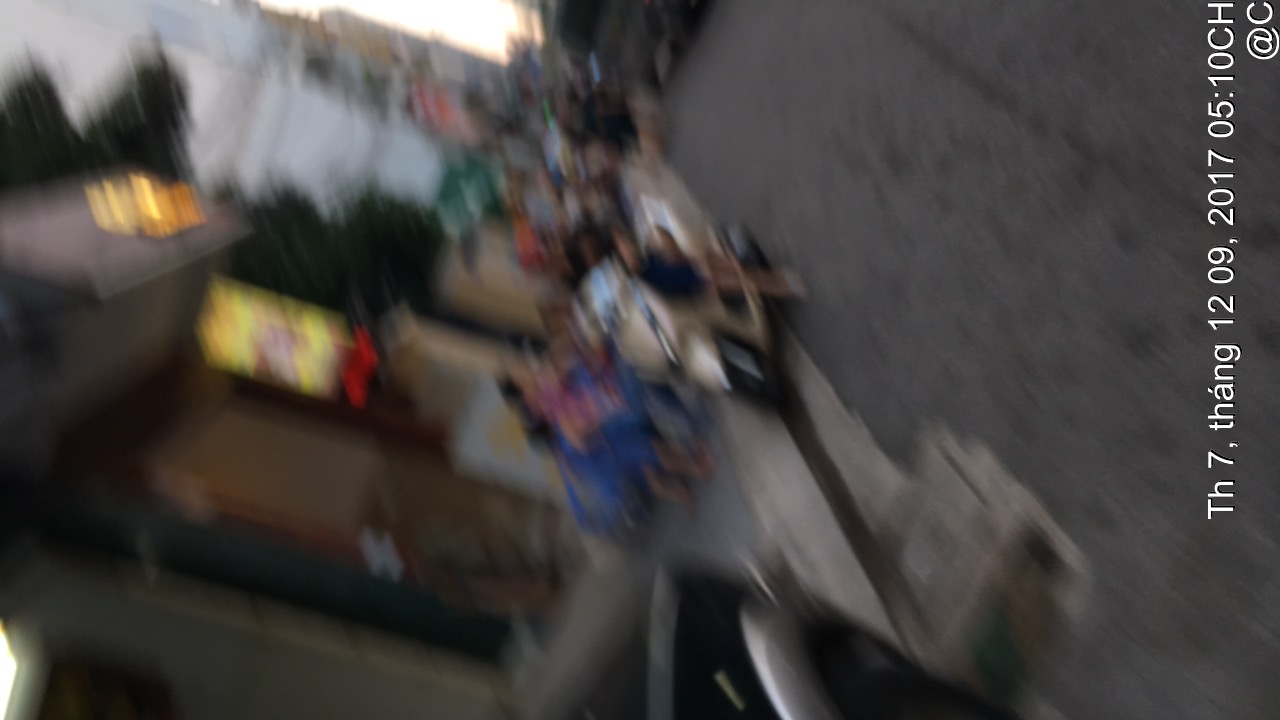The image appears to be a vertical, blurry snapshot, possibly a still from a moving video, taken on a busy street. At the bottom of the image, text reads "TH7 Thang 12-09-2017," suggesting a date format of September 12, 2017. The scene is likely from Vietnam, inferred from the accented text "Thang." The street is bustling with people, with one person clearly visible on a light bronze-colored motorcycle facing the camera. The sidewalk is crowded, and a woman is holding something blue. Additional details include a slanted angle of the photo, hinting at movement, a yellow sign, a brown doorway, and various colors like pink, green, and brown scattered throughout the scene. The camera person appears to be holding something in their left hand, though it is indistinct.